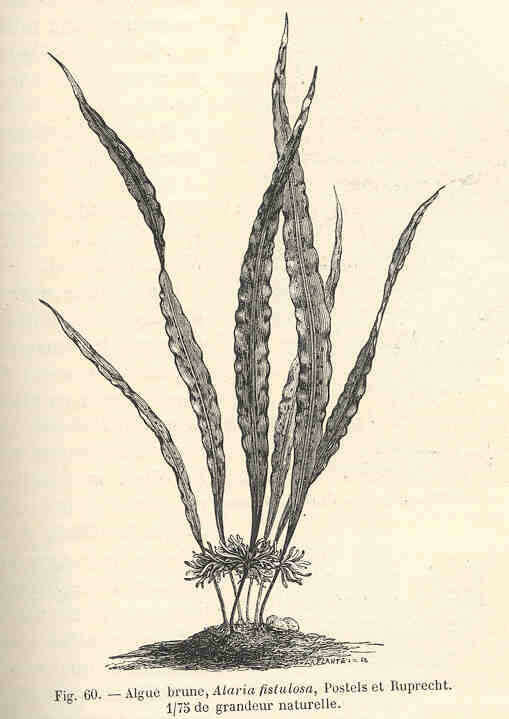This image is a detailed, black-and-white drawing of a plant, likely a scan from an old textbook. The plant features long, tall, skinny leaves that extend upwards, some at slight angles, and stems with flowers that have small petals near their bases. The background resembles yellowish, aged paper, showing wear and slight spotting, adding to the vintage feel. A small pile of grayish dirt sits at the base of the plant. Text at the bottom describes the illustration as "Fig. 60," followed by foreign words, possibly in a European language. Specifically, it mentions "algae brune, Alaria esculenta" and includes a numerical reference "1/75," suggesting it's part of a series. There is an unreadable signature at the bottom, further indicating its archival nature.